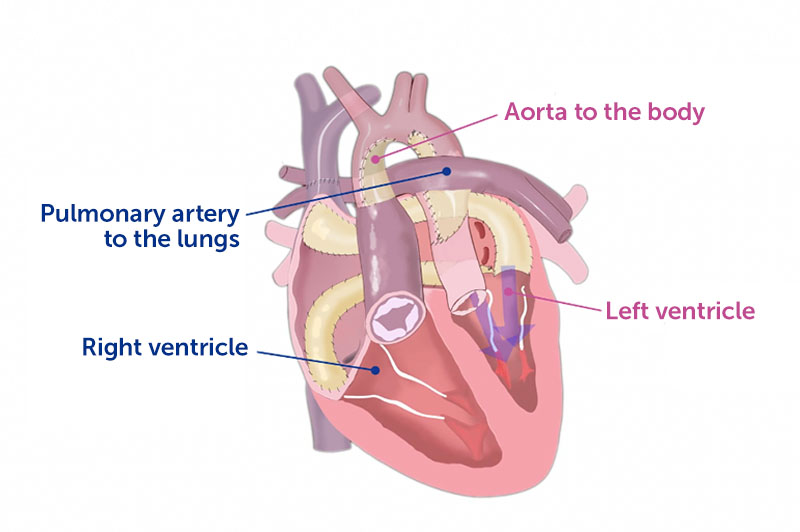A detailed diagram of the human heart on a white background. The heart is primarily illustrated in shades of pink and purple, with some tan hues. The major components are labeled with color-coded text: the "Right Ventricle" is labeled in blue on the left side, the "Pulmonary Artery to the Lungs" is marked in a purple font also on the left, the "Left Ventricle" is noted in magenta text on the right, and the "Aorta to the Body" is labeled in purple at the top. Various lines and arrows in matching colors point to their respective parts, indicating blood flow directions. The diagram includes four labels: right ventricle, pulmonary artery, left ventricle, and aorta. The heart is depicted with vivid details including chambers and multiple connecting tubes, which include both red and dark purple tubes, as well as a distinctive white tube. Although not heavily detailed, the chart provides a basic understanding of the heart’s structure and the location of its key parts.